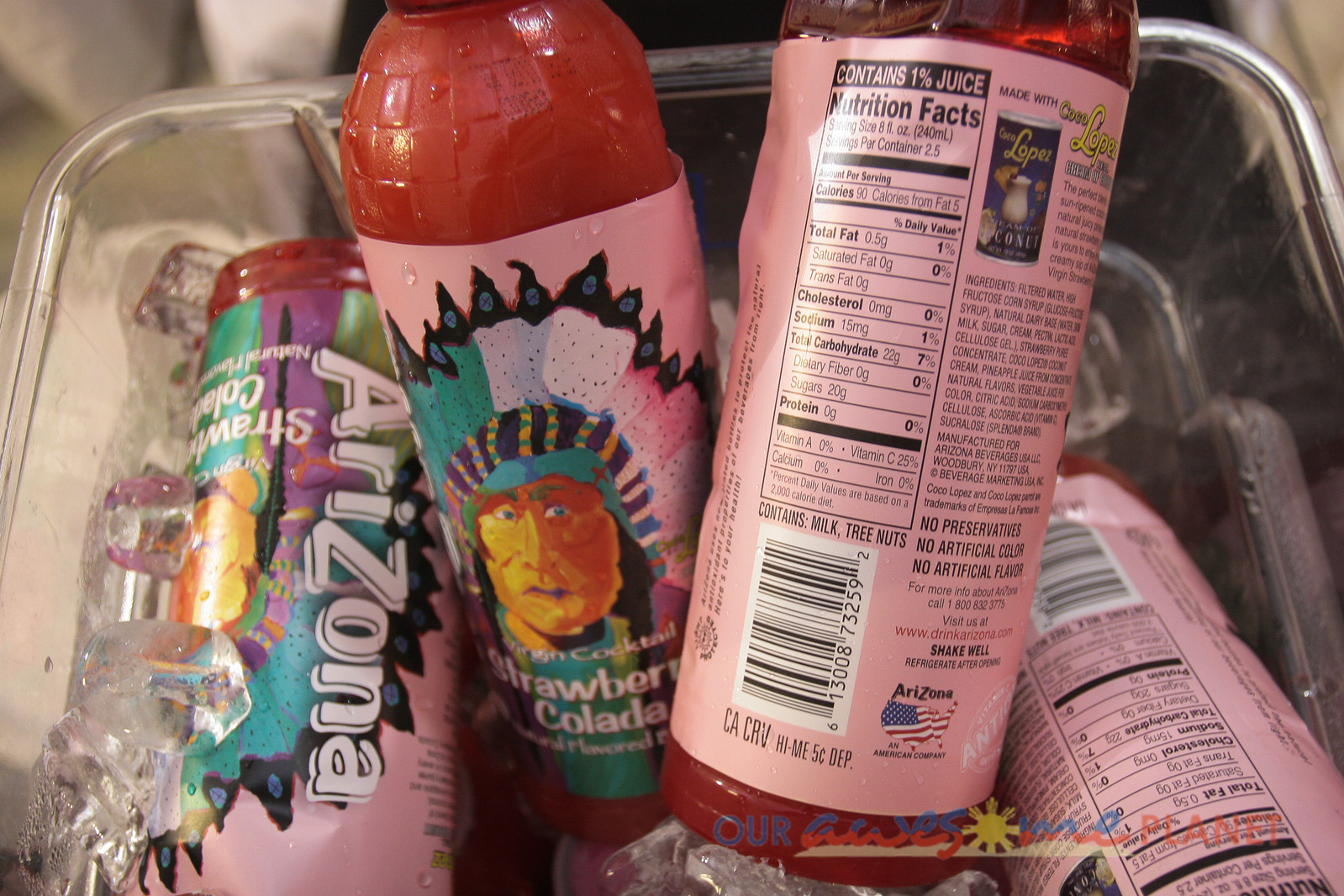This colored photograph offers a top-down view of a clear, square container, presumably a tray, holding four bottles. The most visible bottle features a label with a vertical "Arizona" branding by the Arizona Tea Company, printed in pink. The partial label also indicates "strawberry" as part of its flavor description. A second bottle's front label displays a detailed color illustration of a traditional Indian chief wearing a headdress, with "strawberry colada" clearly printed below the image, identifying the flavor. The third bottle is turned, showing the back of the label with nutrition facts and a barcode. Although the text is too small to read, it's positioned beneath a column of smaller, unreadable print. The fourth bottle also shows its barcode and partial nutrition facts.